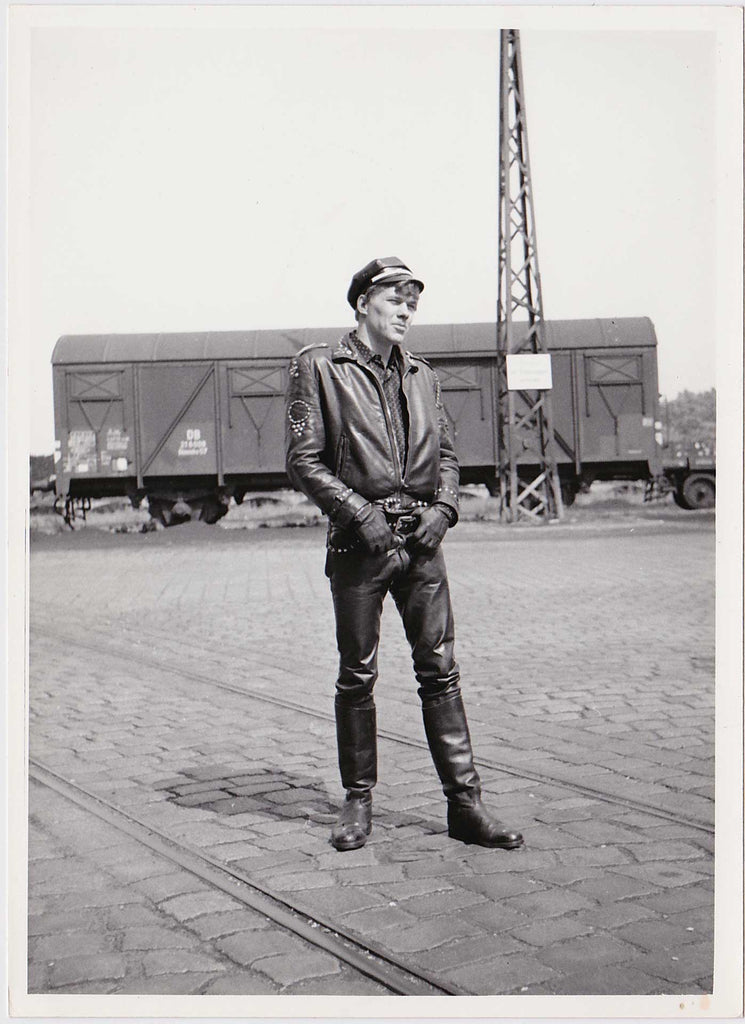In this striking black-and-white photograph that seems to harken back to the 1940s or 1950s, we see a tall, clean-shaven Caucasian man dressed entirely in leather, giving off a rebellious, Marlon Brando-esque vibe. The man is outfitted in a black leather jacket with studded designs, a patterned collared shirt beneath, black leather pants, knee-high black boots, leather gloves, and a distinctive leather cap that resembles a police officer's hat. He stands confidently with his hands on his waist, possibly resting on a belt buckle, as he looks off into the distance. 

The setting appears to be an old cobblestone street with tram tracks running along it, suggesting a bygone era when these tracks were likely in use. In the background, there is an abandoned train car and a towering radio or telegraph structure, adding to the photograph's nostalgic ambiance. The overall scene captures the essence of a lone biker posing against an industrial backdrop, creating a timeless image that blends rugged individualism with a touch of vintage cool.